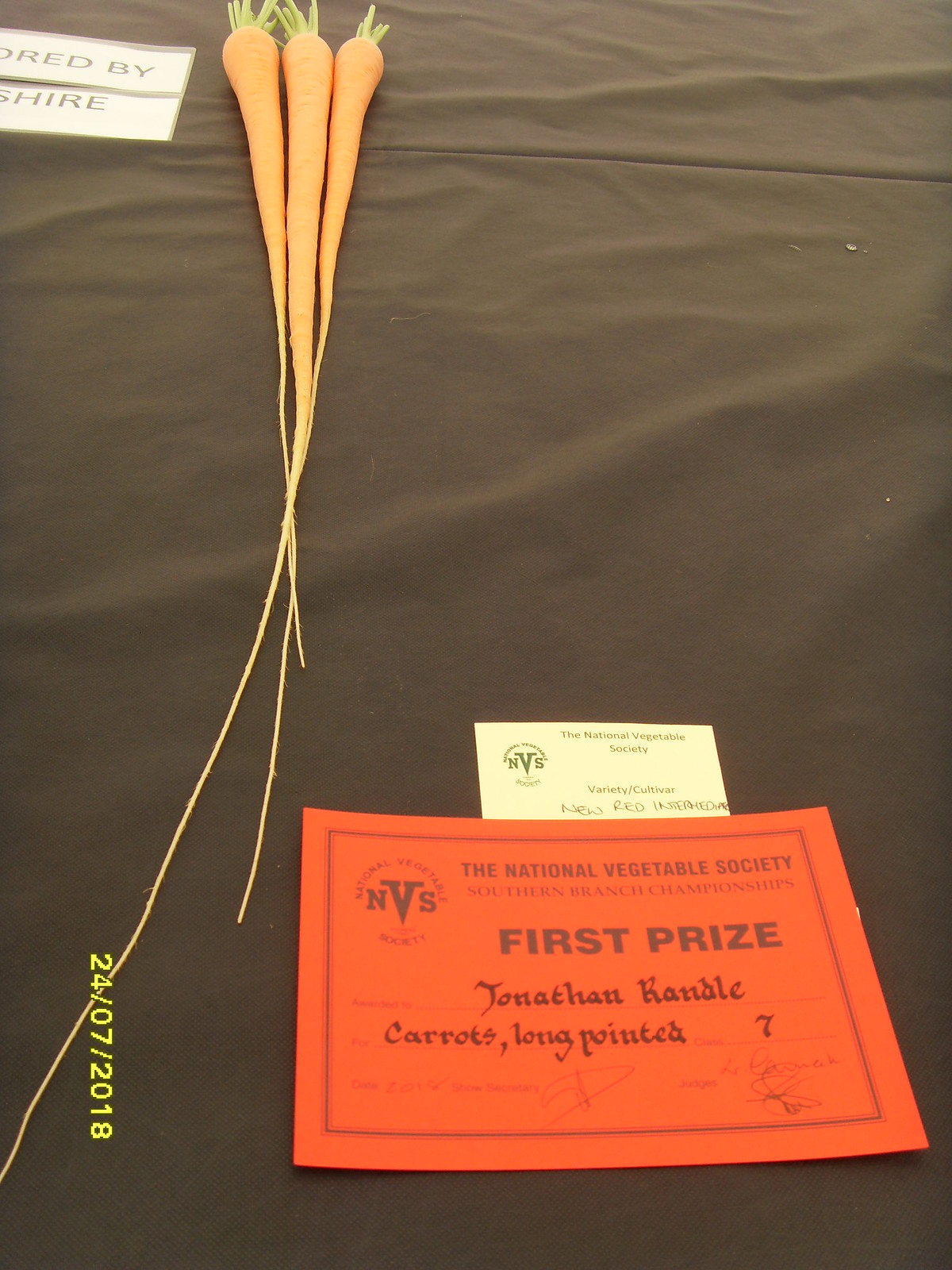This photograph features three exceptionally long, prize-winning carrots placed diagonally on a black tablecloth. The carrots, with their leafy tops trimmed, extend across the upper left corner of the image. Supporting their prestigious status, an orange placard at the bottom of the photograph proudly proclaims "First Prize," awarded to Jonathan Randall for his "Long Pointed" carrot variety. Adjacent to this, a red sign from the National Vegetable Society (NBS), Southern Branch Championships confirms the award, bearing their logo and details of the victory. Additionally, a white business card, also featuring the NBS logo, is partially visible above the placard. In the lower left corner of the image, yellow text displays the contest date as 24-07-2018. A portion of another text element reading "Redshamshire" can be seen in the top right corner, although partly obscured.